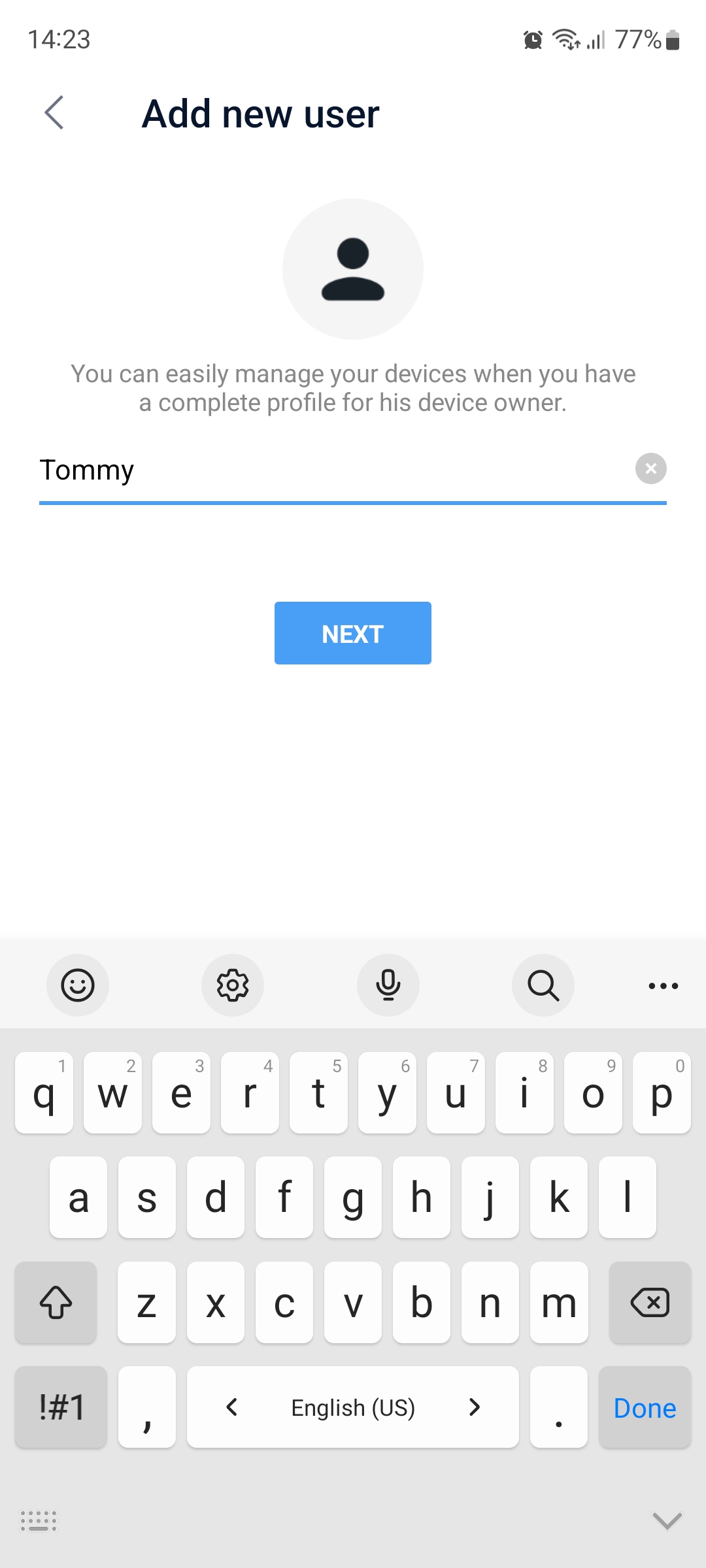A detailed screenshot of a smartphone's user interface captured at 2:23 AM displays a battery level at 77% and a strong network signal, all set against a crisp white background. At the top of the screen, there's a left-pointing arrow followed by the text "Add New User." Below this, a prominent gray circle contains an icon of a person, signifying the user profile section. A helpful instruction beside this icon informs users that they can "easily manage your devices when you have a complete profile for the device owner." Further down, a blue bar highlights the name "Tommy," indicating the user's profile. Towards the bottom, a blue button labeled "Next" in white text invites the user to proceed with the setup. Beneath all these elements, the virtual keyboard is visible, suggesting it's ready for input.